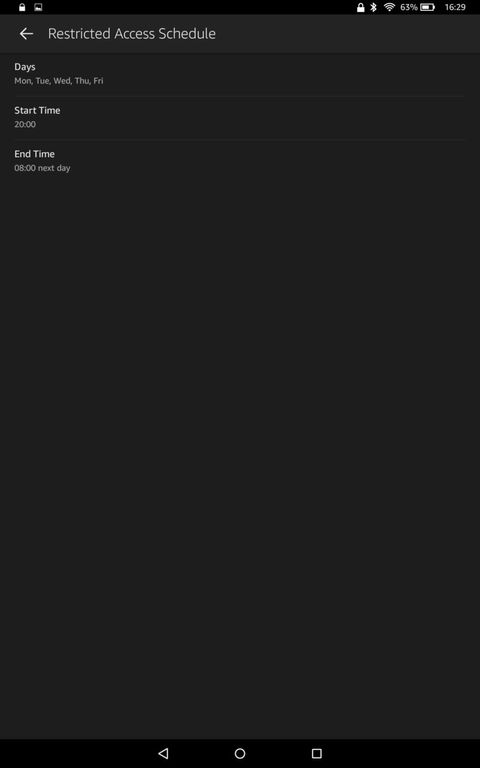The image is a screenshot taken from a cell phone. At the top left corner, two small cell phone icons are visible. On the top right corner, there are several status indicators: a Bluetooth icon, a Wi-Fi icon, and a battery percentage reading 63%. The current time displayed is 16:29. Just below this, aligned to the left side, is a backward-facing arrow, followed by the text "Restricted access schedule" in white font.

The main content of the screen is divided into three categories stacked vertically: "Days" at the top, followed by "Start time" in the middle, and "End time" at the bottom. Each category is presented on a black background, providing a stark contrast for readability. 

At the very bottom of the screen, three cell phone navigation icons are displayed. The left icon is a sideways triangle, the middle icon is a circle, and the right icon is a square. These icons are also white and set against a slightly darker black background, ensuring they stand out for easy navigation.